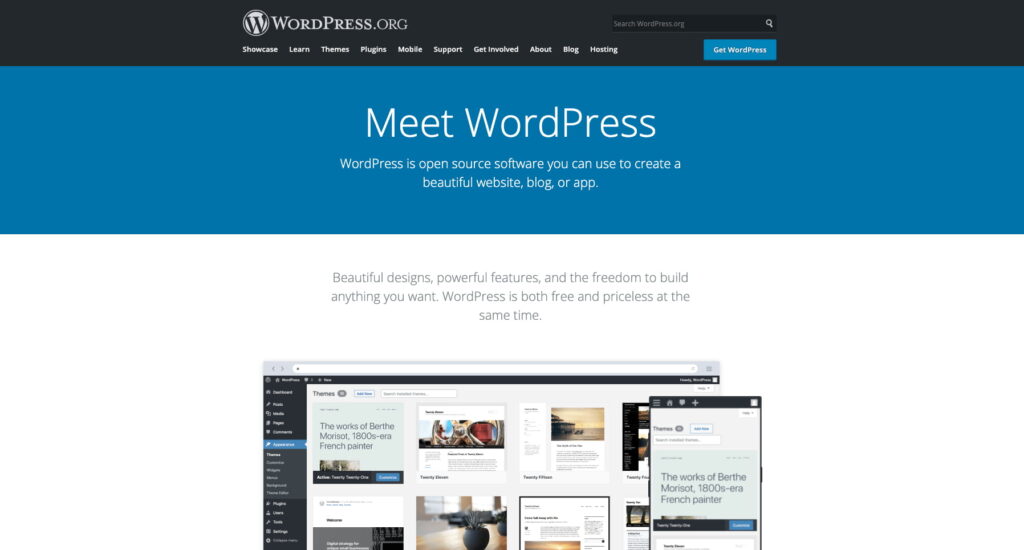The home page of WordPress.org is presented in a clean and structured layout with notable symmetry and distinct color borders. The page features black, blue, and white borders with a two-inch gap on the left and right sides, concentrating the main content at the center. 

At the top, a slender black border about an inch thick frames the header. Inside it, against a white background, is a prominent white circle containing a black "W" logo, encircled by a black border. To the left of the logo, "wordpress.org" is displayed in bold white lettering. Following a two-inch gap to the right is a sleek black search bar with the text "Search wordpress.org" in white and an accompanying search icon on the right side.

Directly below the header, a blue tab is visible with "Get WordPress" inscribed in white. Beneath the WordPress logo, a concise navigation menu in small white text includes links such as "Showcase," "Learn," "Mobile," "Support," "Get Involved," "About," "Blog," and "Hosting," extending horizontally from left to right.

In the primary content area, a blue section prominently features the phrase "Meet WordPress" in large white letters. Below, a detailed description reads, "WordPress is open source software you can use to create a beautiful website, blog, or app." Continuing downward into the white section, a concise, impactful message is displayed in black text: "Beautiful designs, powerful features, and the freedom to build anything you want. WordPress is both free and priceless at the same time."

An out-of-focus image showcasing the WordPress app is situated further down, adding a visual element to the text-centric layout, illustrating the practical application and user interface of the WordPress platform.